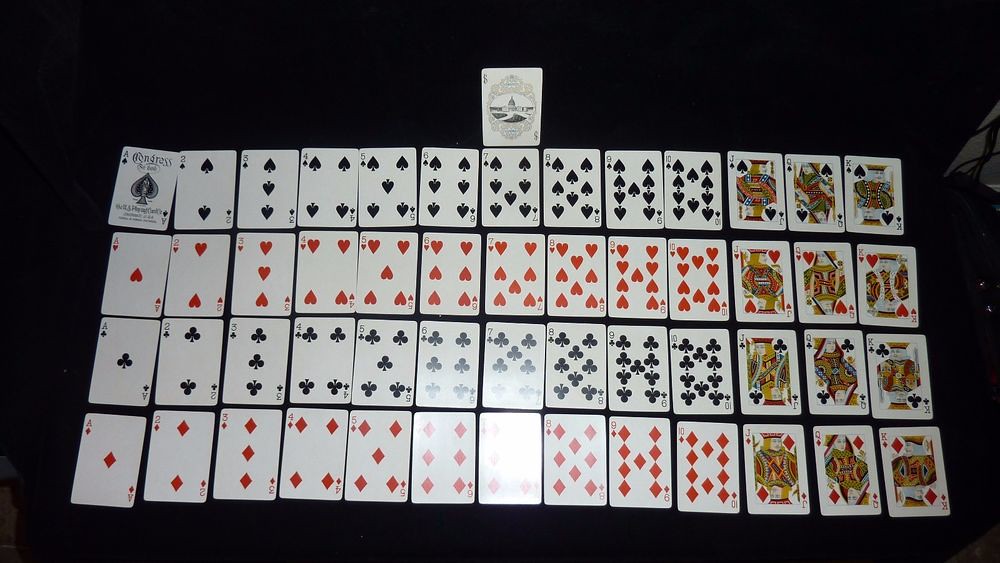A meticulously arranged full deck of playing cards is displayed in four horizontal rows against a murky, black background. The light source is glaringly harsh, emanating from above and beaming down with intense brightness at the bottom center of the image, almost to an uncomfortable level. At the very top, a partially visible white rectangular outer box or sleeve with an indistinct black design seems to float above the spread-out cards.

The first row showcases the spades suit in perfect sequence, starting from the Ace of Spades, which prominently displays the card manufacturer's name and other details, followed by the series 2 through 10, and concluding with the Jack, Queen, and King of Spades.

Following below, the second row features the hearts. From the Ace of Hearts, the row continues in numerical order up to 10, followed by the face cards: Jack, Queen, and King of Hearts.

The third row mirrors the format with the clubs. Starting with the Ace of Clubs, the sequence proceeds through the numbers 2 to 10 and finishes with the Jack, Queen, and King of Clubs.

The bottom row, which is marred by the severe glare, contains the diamonds. Beginning with the Ace of Diamonds, it follows with the cards 2 through 10, and ends with the Jack, Queen, and King of Diamonds.

To the very right edge of the photograph, a faint glimmer of light reveals a hint of an object, potentially an electrical cord, though it remains mostly undefined.